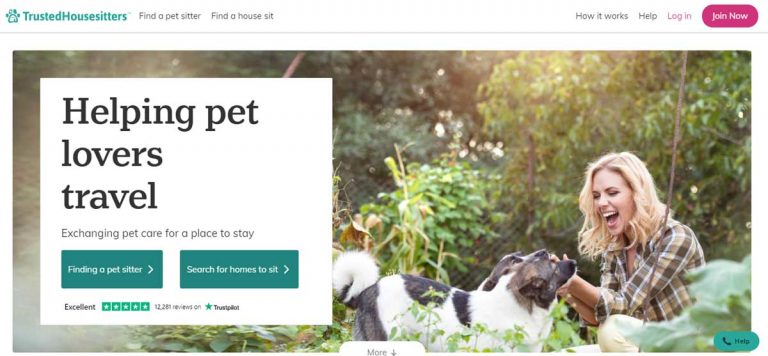The image depicts a clean and minimalist website design for a service called "Trusted House Sitters." The primary focus of the page is a large, high-quality photograph that dominates the screen. It features a blonde woman with short hair petting two dogs, one mostly black and white, and the other with a mix of black and brown on its face. They appear to be in a lush garden setting, possibly a backyard, with trees in the background.

The header of the page prominently displays the text "Trusted House Sitters" in turquoise. Below it are navigation links: "Find a Pet Sitter" and "Find a House Sitter." To the right, additional links read: "How it Works," "Help," "Log In," and a clearly visible pink button labeled "Join Now."

On the left side of the image, there is a white text box that reads: "Helping pet lovers travel by exchanging pet care for a place to stay." Below this text are two green buttons: "Find a Pet Sitter" and "Search for Homes to Sit."

At the bottom of the page, a Trustpilot score is displayed, indicating an "Excellent" rating with a total of 12,281 reviews.

Overall, the page exhibits a simple yet effective design, characterized by its clean layout and easy navigation, making it user-friendly and visually appealing.